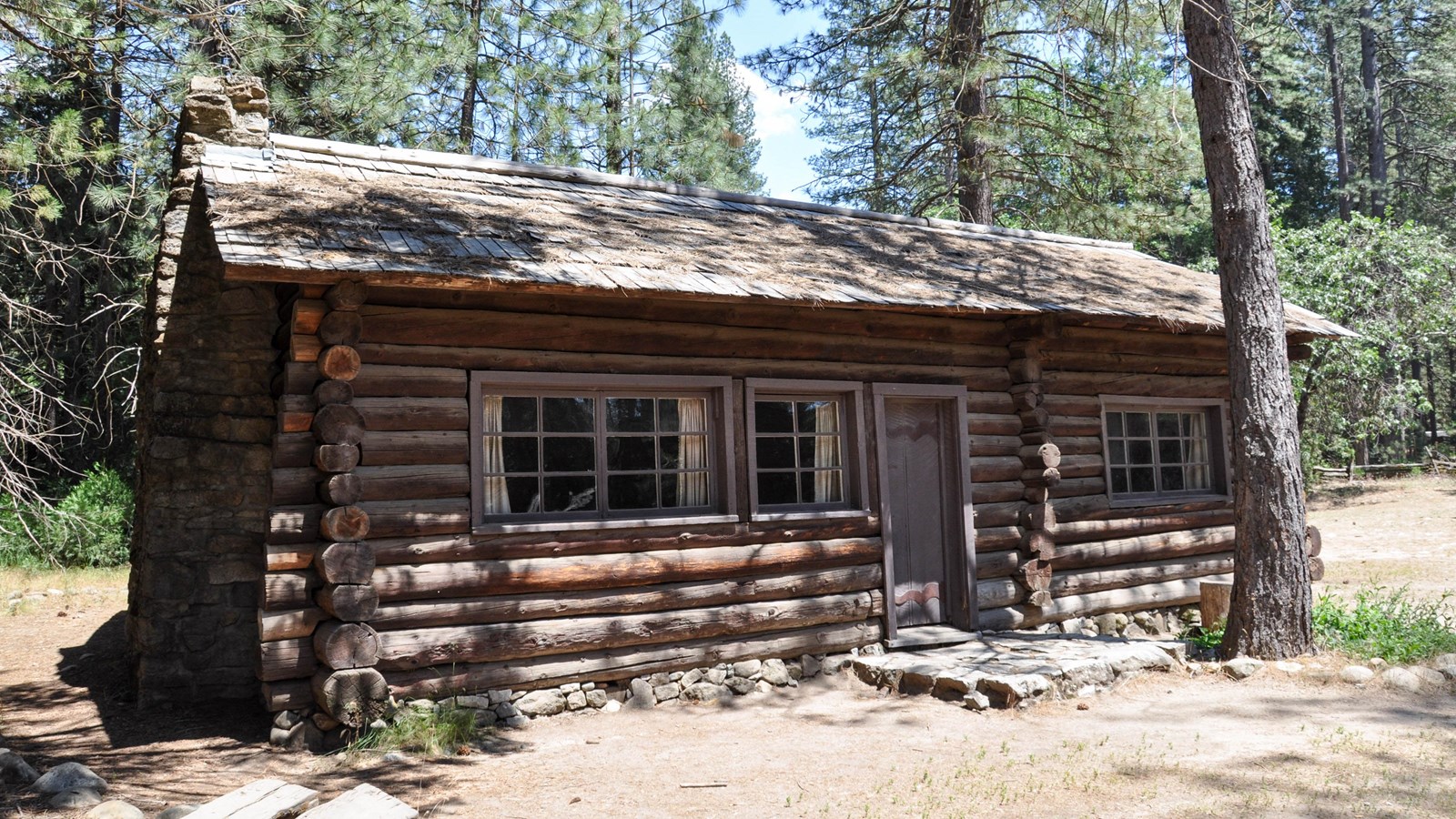The image depicts a small, rustic log cabin that appears to be handmade. The cabin features two sections that suggest it may contain two separate rooms. The structure is crafted from cross-hatched logs, with their ends extending at right angles at the corners. Its roof is covered in wooden shingles and is littered with pine needles, indicating a forested setting around it, with pine trees nearby. The entrance showcases a modern wooden door accompanied by three sections of glass windows – two wider ones and a narrower one adjacent to the door. Despite its old rustic design, it remains uncertain if the cabin is an antique, newly constructed, or restored, though its materials and construction suggest a more recent build styled traditionally. A stone-built chimney is attached to the left side of the house, and rocks are piled at the base with a square stone and mortar structure serving as a stoop in front of the door. There is some observable damage on the rooftop, and the entire cabin exudes a quaint, historical charm amidst its verdant forest surroundings.